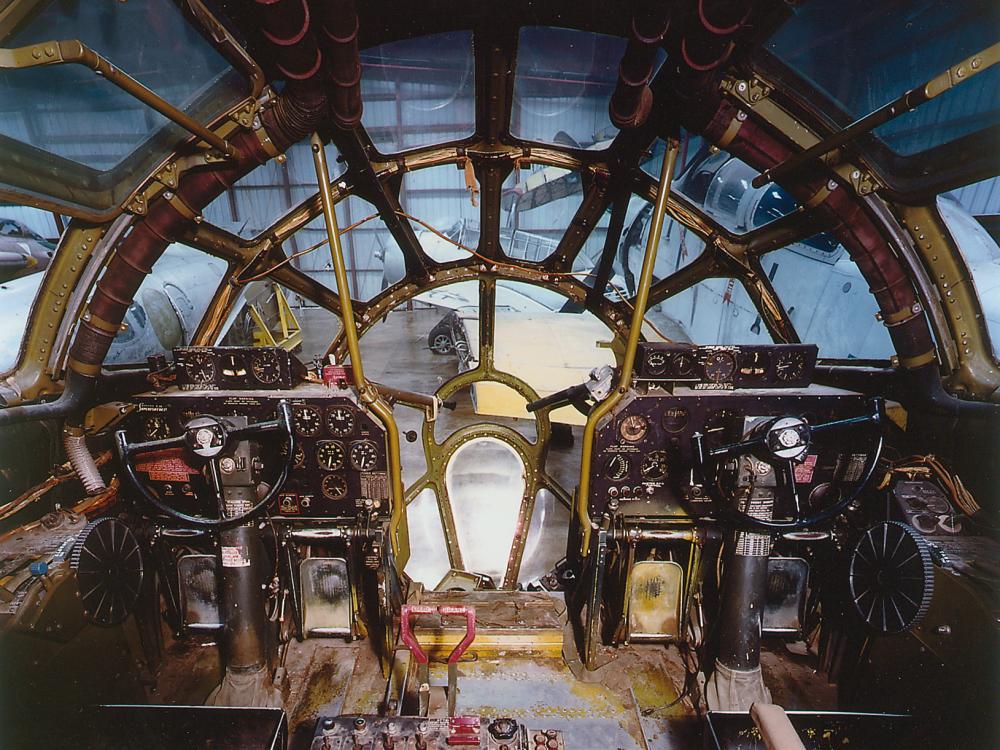The image depicts the dark and weathered cockpit of what appears to be a vintage World War II bomber airplane, likely housed in a museum or storage hangar filled with other aircraft. The cockpit is framed with strong, yellow-trimmed steel and encompasses a panoramic array of rounded windows, some of which are pane-less or made from heavy-duty glass or plastic. The front of the cockpit features two widely separated pilot seats, although the chairs themselves are missing. A narrow passageway between the pilot positions likely leads to a nose gunner's position, typical of a bomber. The interior is adorned with analog controls, including two half-moon, black steering wheels, numerous dials, buttons, gauges, and red and yellow tubes and handles. The floor is tan with some steel plates and mold patches, suggesting long-term disuse. The trim within the cockpit is primarily gold, brown, and black, contributing to its historic and rustic appearance. Overall, the cockpit scene is rich in mechanical detail, evident in the intricate array of knobs, gears, and pipes, enhanced by the vivid contrasts of red, yellow, and black against the worn metal backdrop.